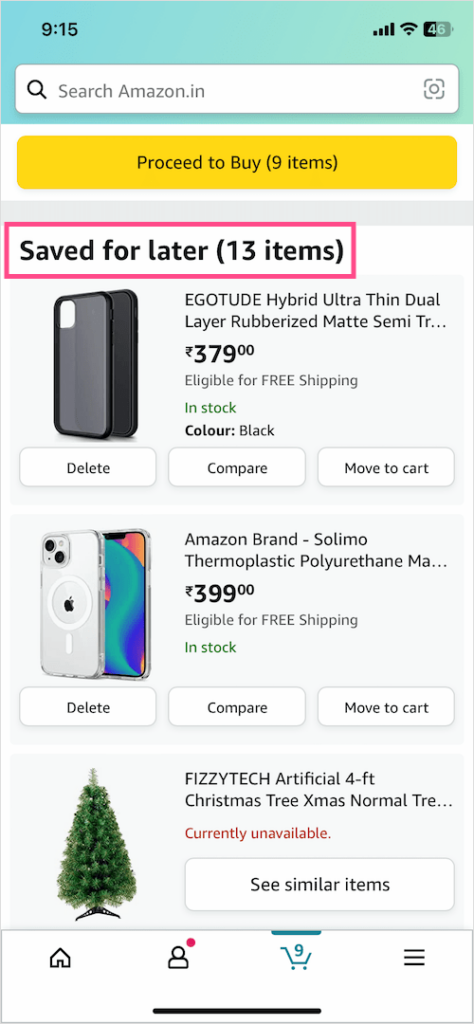Screenshot of the Amazon.in shopping cart page, likely from the Indian version of Amazon, displaying items in Indian Rupees (₹). The top of the screenshot shows the search bar with the text "search amazon.in" indicative of the Indian market. Below this, there's an actionable yellow button labeled "Proceed to Buy (9 items)" and a red or pink box highlighting the "Save for Later (13 items)" section.

In the "Save for Later" section, the focal point includes a variety of products, such as:

1. **Ego to Hybrid Ultra-Thin Dual Layer Rubberized Matte Semi...** (partial description due to cut-off)
   - Price: ₹379
   - Status: In stock, eligible for free shipping
   - Options: Delete, Compare, Move to Cart

2. **Amazon Brand Solimo Phone Case (Thermoplastic Polyurethane Material)**
   - Price: ₹399
   - Status: In stock, eligible for free shipping
   - Options: Delete, Compare, Move to Cart

3. **Fizzy Tech Artificial 4 Feet Christmas Tree**
   - Status: Currently unavailable
   - Note: Likely been in the cart for an extended period
   - Option: See similar items for alternative purchases

At the bottom of the screenshot, the navigation bar includes icons for Home, Personal Profile, Basket, and Menu options, common in mobile apps for easy navigation.